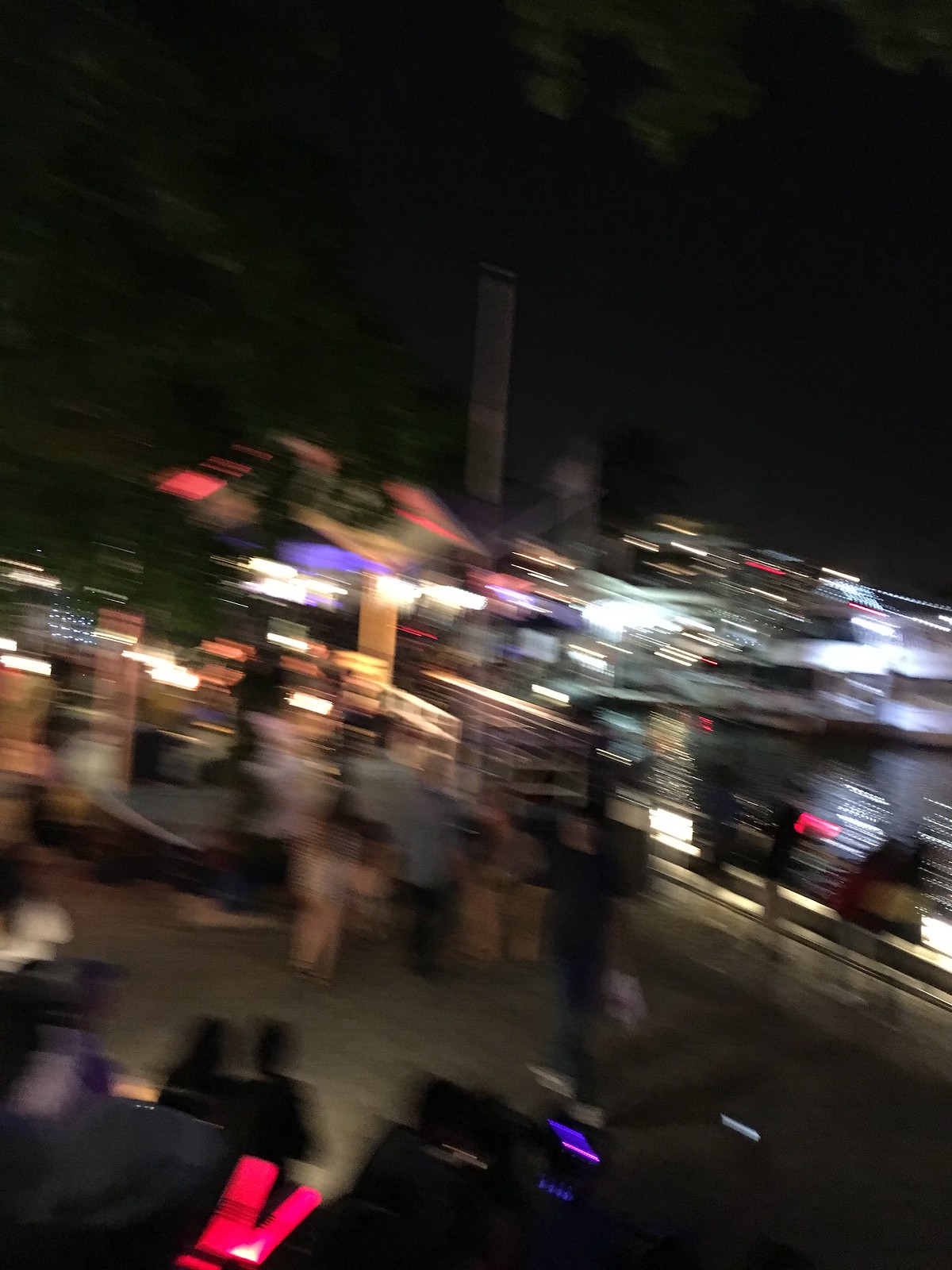This is a color photograph taken at night, likely depicting an outdoor event such as a concert, festival, or carnival, given the presence of people and numerous lights. The scene is notably blurry, with streaks and light trails that suggest movement. Toward the middle of the image, a group of people of varying sizes, including children and adults, are visible, possibly waiting in line or seated on benches. In the bottom left corner, an individual holding red pen lights stands out amidst the blurriness. The right side of the photograph reveals a body of water, framing the gathering. There are also suggestions of camera or computer equipment with blue and black screens on the scene, adding to the electronic ambiance. The background of the image hints at green trees, though they are shrouded in darkness. Overall, the photograph captures a dynamic and lively nighttime event, albeit with a significant amount of motion blur.